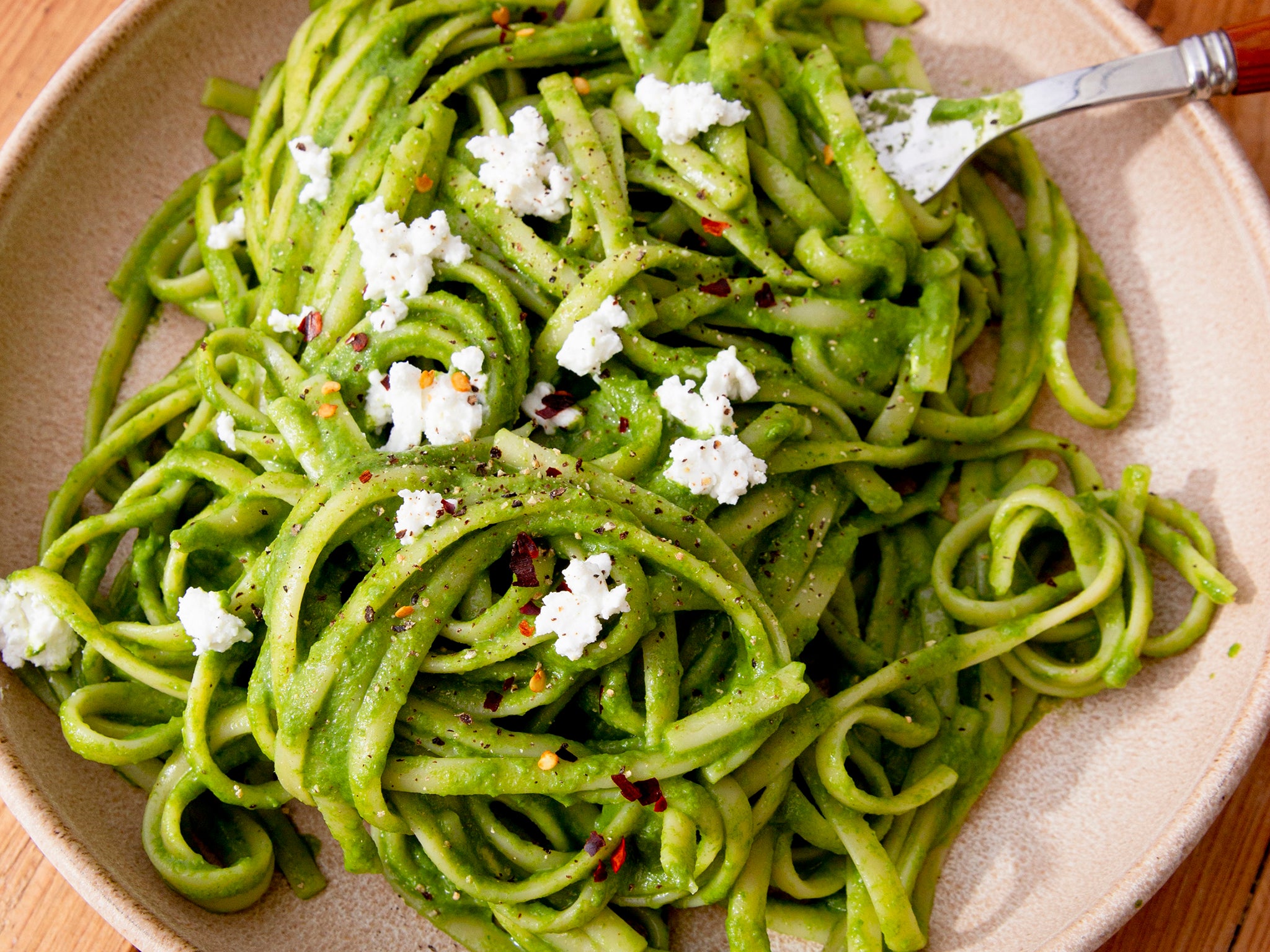The image showcases a beautifully arranged dish of green zucchini fettuccine, elegantly presented on a handmade, light brown ceramic plate. The fettuccine is flat and lies intertwined, adorned with an assortment of seasonings, including visible red and yellow spices, crushed red pepper flakes, and what is likely salt and pepper. Scattered across the pasta are crumbles of white cheese, presumably feta. The dish is served without any sauce, allowing the spices and cheese to take center stage. A silver fork with a wooden handle is partially inserted on the right side of the plate, emphasizing the act of dining. The plate rests on a walnut-colored wooden table, adding a rustic charm to the composition. The close-up nature of the photograph highlights the intricate details of the dish and the artisanal quality of the pottery, creating a warm, inviting scene.